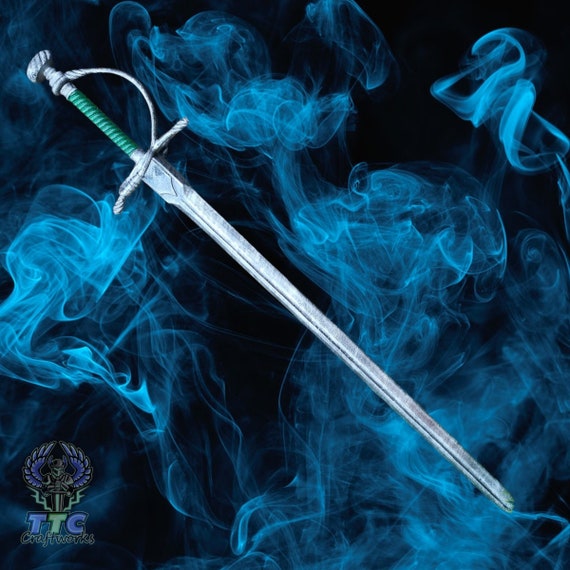This is a highly detailed image showcasing an ancient or old sword positioned diagonally from the upper left to the bottom right corner. The sword, which is long and slender, has a ridge running down the center of its silver blade. It features a handle wrapped in a green material and a metal loop extending from the start of the blade to just before the knob of the handle. The detailed background combines a completely black setting with swirls of bright cyan blue smoke, creating an ethereal effect. In the bottom left corner of the image, there is a symbol resembling wings or horns, accompanied by the letters "TTC" and the word "Craftworks," indicating the maker of this impressive weapon.